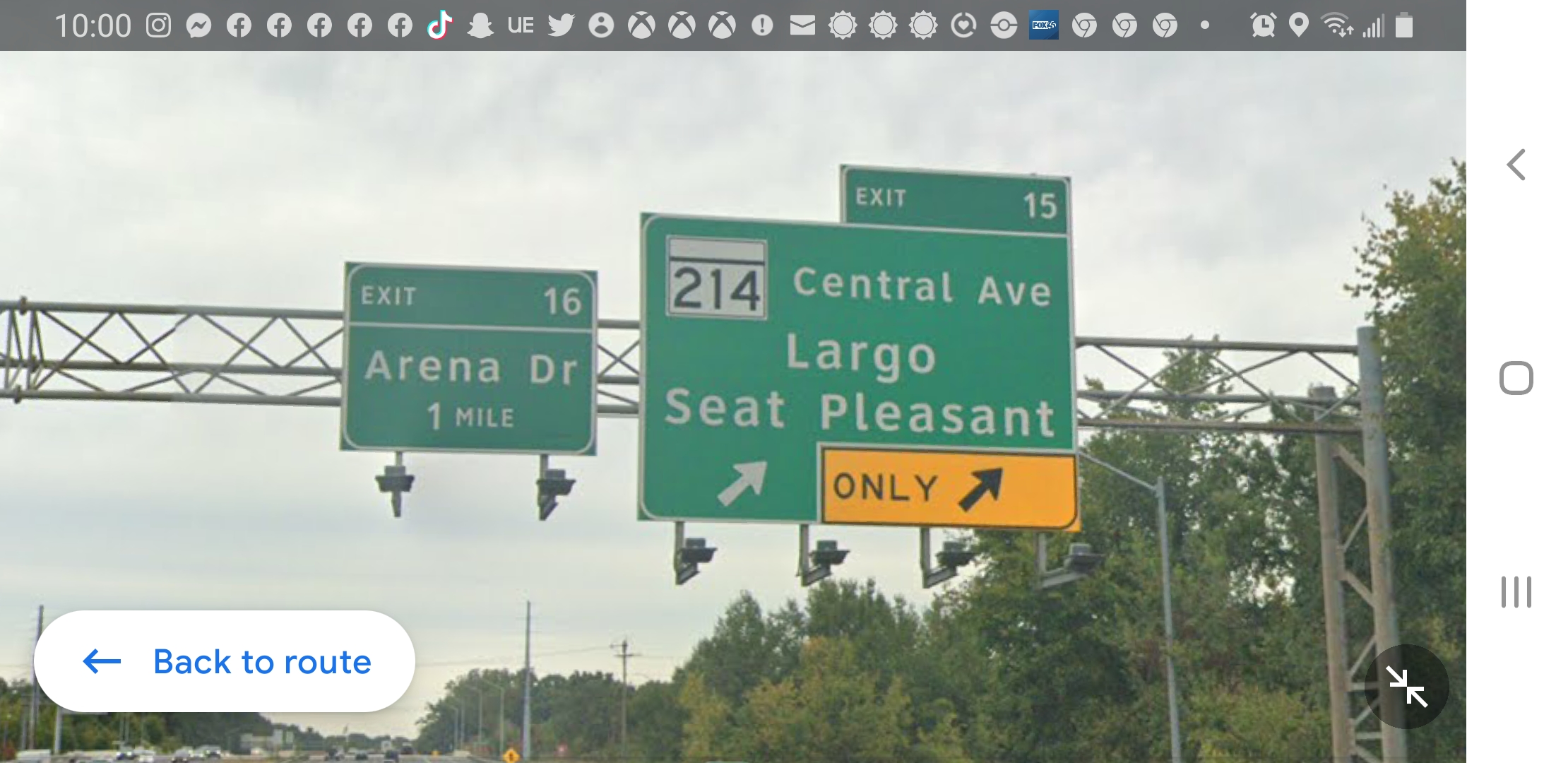The photograph is a detailed, color image depicting a pair of highway signs suspended from a metal support structure. The left sign is green with white lettering, indicating "Exit 16, Arena Drive, 1 mile." The right sign is larger, also green with white lettering, and reads "Exit 15, 214 Central Ave, Largo, Seat Pleasant" with a diagonal white arrow pointing to the upper right. Below this sign, a yellow section with a black arrow bears the word "Only," also pointing diagonally upward to the right. In the bottom left corner of the image, there is a white oblong label that says "Back to Route." The background features a light blue-grayish sky and is filled with tall trees, both on the right side and extending into the bottom left of the image, where additional power poles and parts of the freeway can be seen, showing the interconnected infrastructure. The top of the image is overlaid with a black bar displaying multiple digital indicators, including icons for battery life, signal strength, Wi-Fi, GPS, an alarm clock, and notifications from apps such as Facebook, TikTok, Snapchat, Uber Eats, Twitter, and Xbox, which suggest the image was captured from a mobile device screen.